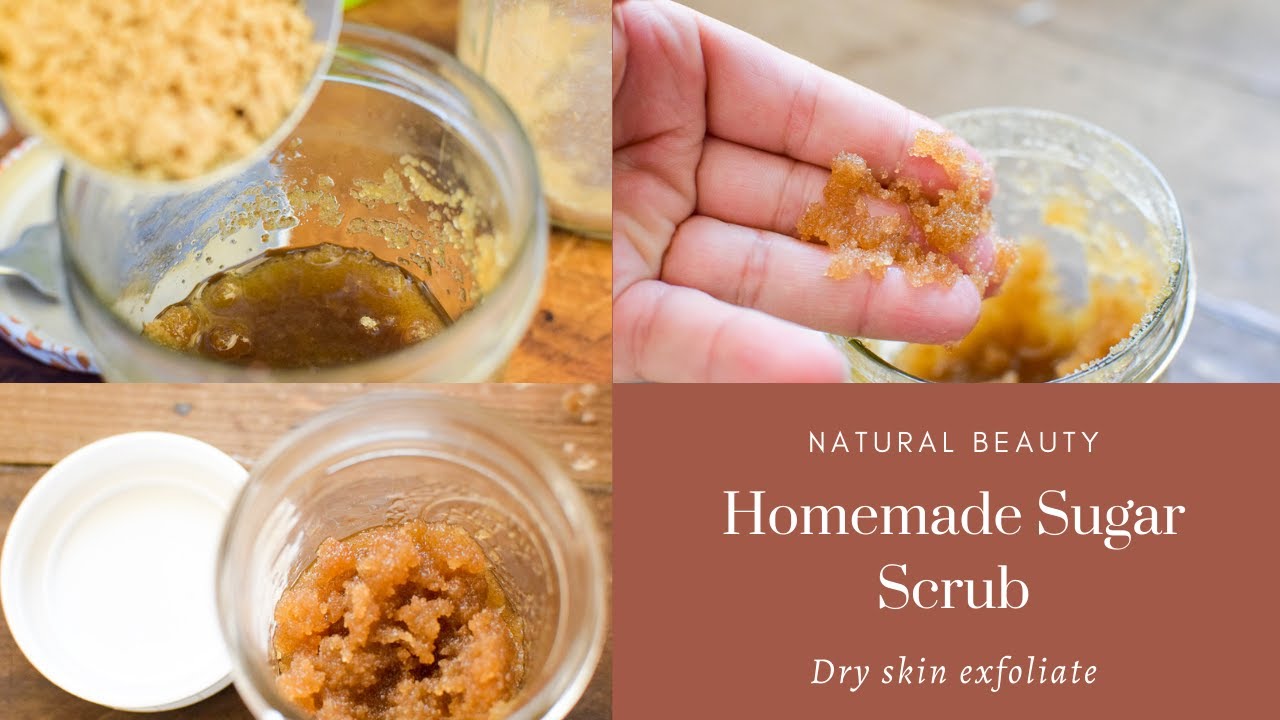This is a detailed four-panel advertisement or magazine page presenting a "Natural Beauty Homemade Sugar Scrub" for dry skin exfoliation. The panels are arranged in a landscape orientation, with three panels dedicated to representing the sugar scrub preparation and usage, and the fourth panel featuring promotional text. 

In the upper left corner, there is a clear glass jar partially filled with a syrupy, golden-brown mixture. Brown sugar is about to be poured into this jar, which sits on a medium-colored wooden surface. The jar has a twist-off white lid resting next to it.

The upper right panel shows a close-up of a left hand holding a small amount of the sugar scrub mixture. The scrub in this image appears textured, resembling oily brown sugar. The background includes parts of the jar and the wooden surface.

In the lower left panel, the glass jar is seen again, this time filled with the mixed scrub, displaying a uniform, clumpy consistency. The white lid is placed next to the jar on the wooden surface, emphasizing the homemade nature of the product.

The lower right panel features a brown background with white text reading "Natural Beauty Homemade Sugar Scrub Dry Skin Exfoliant," formatted like a business card or label, adding a professional touch to the homemade product.

Overall, this advertisement captures the step-by-step process and effectiveness of the homemade sugar scrub, highlighting its natural ingredients and benefits for dry skin.